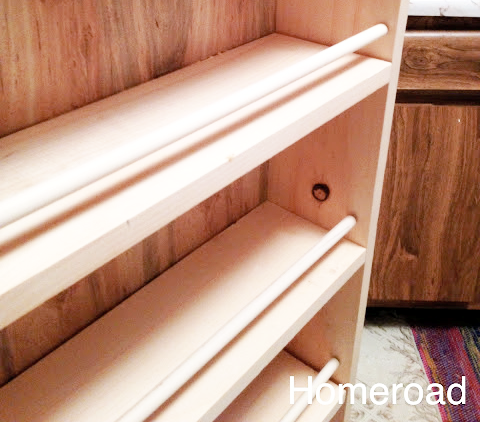This indoor photograph showcases a light-colored wooden spice rack mounted inside a darker wooden cabinet door. The spice rack features three levels supported by a vertical board on the right, with each shelf equipped with a small, round wooden dowel placed above the front edge to prevent items from falling out. The cabinet and drawers to the right are a darker wood, and the stone floor is partially covered by a red carpet visible in the bottom right corner. Superimposed in white text at the bottom right of the image is the word "HOMEROAD." The photograph primarily focuses on highlighting the spice rack, which appears to be a newer addition to the cabinet setup.